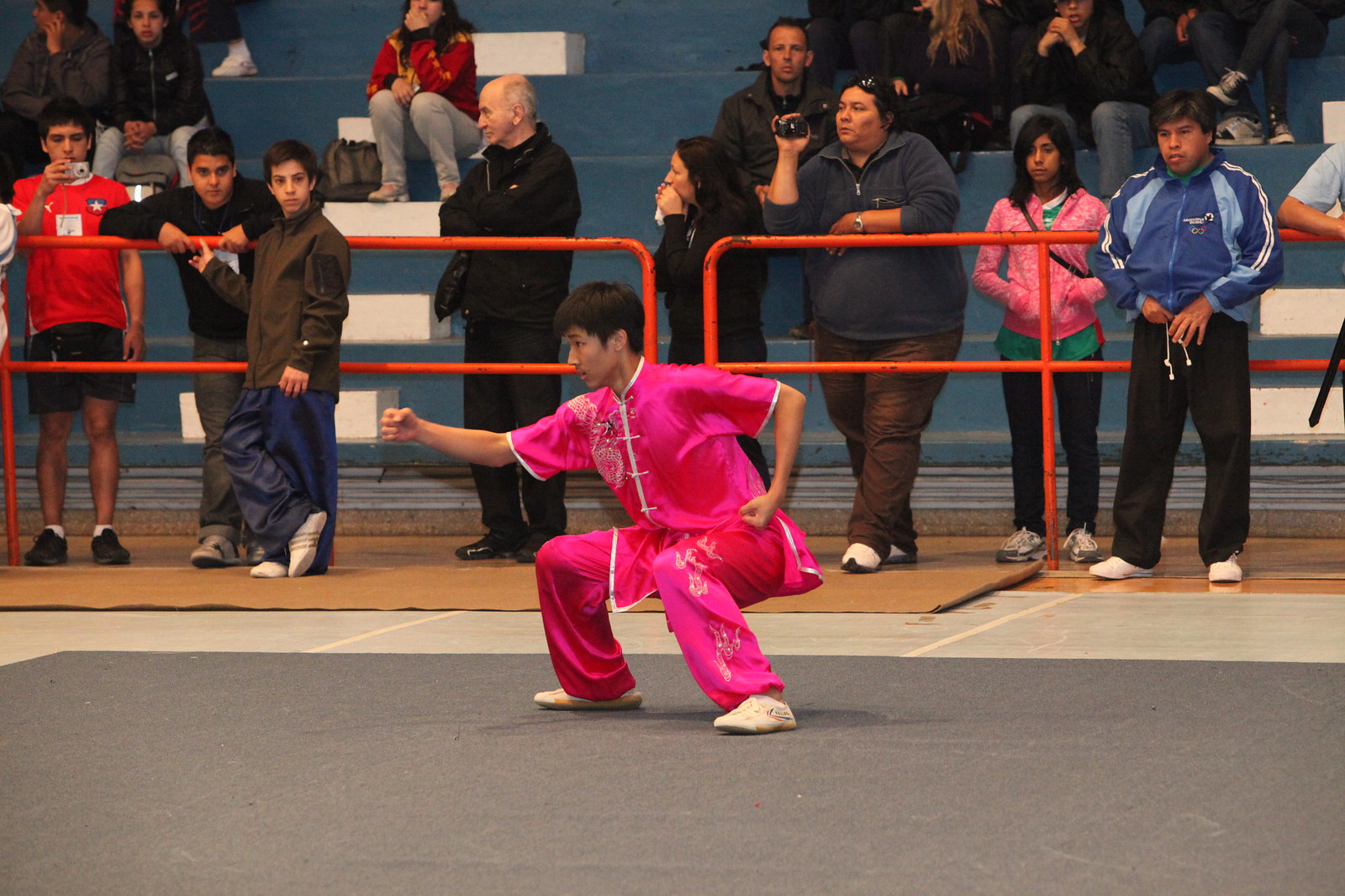In the photograph, a slim, young Asian man is captured mid-performance, striking a dynamic karate pose on a gray mat inside a gymnasium. He stands with one arm on his hip, clenched in a fist, and the other arm extended outward toward the crowd, also in a fist. Emphasizing his form and tradition, he is adorned in a formal, pink outfit that suggests traditional Asian attire, possibly indicative of a Taekwondo demonstration. The scene is framed by orange bars that act as a fence, behind which a mixed audience of standing and seated spectators watch intently. Among them, a boy captures the moment with his camera, while a woman records the event with a video camera. Other onlookers include a woman with sunglasses resting on top of her head and another with a purse beside her. The crowd, composed of various individuals, adds to the lively atmosphere of this culturally rich and performative display.